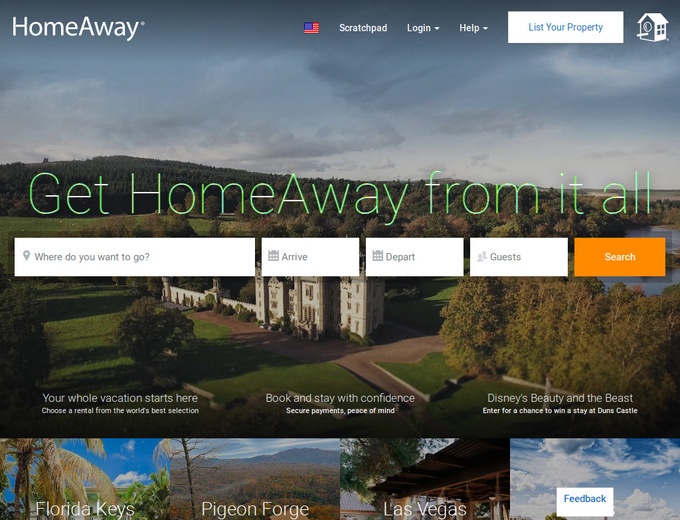This image is a cropped screenshot of a section of the HomeAway desktop web page, which features an aerial view of a picturesque castle nestled within dense woods as its background photo. 

At the top left corner, the HomeAway logo is prominently displayed in large white letters. Moving to the top right, there is a horizontal menu listing various categories, a prominent white bar encouraging users to "List Your Property," and a small birdhouse icon, which is centrally positioned over the scenic photo background. Overlaying the background, a bold white text message reads "Get Home Away From It All."

Beneath this message and aligned to the left, is a large text box prompting the user with "Where do you want to go?" in small gray letters. Adjacent to this, the interface includes two smaller text boxes labeled "Arrive" and "Depart," both featuring calendar icons for date selection. To the right of these boxes is another small box labeled "Guests," and at the far right is a striking orange "Search" button.

Occupying the bottom portion of the image, there are four square-shaped categories, each adorned with a photo background and white text overlays. The categories from left to right read: "Florida Keys," "Pigeon Forge," and "Las Vegas." The name of the fourth category is partially obscured by a white feedback box, making it unreadable.